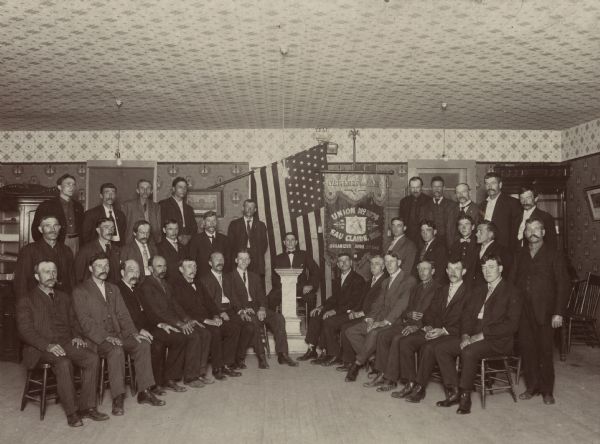This black-and-white photograph, seemingly taken pre-1940s based on the style of clothing, captures a group of men, some standing and some seated, all with short hair and several sporting handlebar mustaches. They are dressed in darker-colored suits. The focal point of the image is a man seated behind a podium at the center, with an American flag positioned behind him. The setting is an intricately decorated room, featuring wallpapered walls and ceiling. A reflection of the camera flash is noticeable on the back wall, while overhead light fixtures hang from the ceiling. The room has a visible wooden floor, and all the men are directed at the camera with intense gazes.